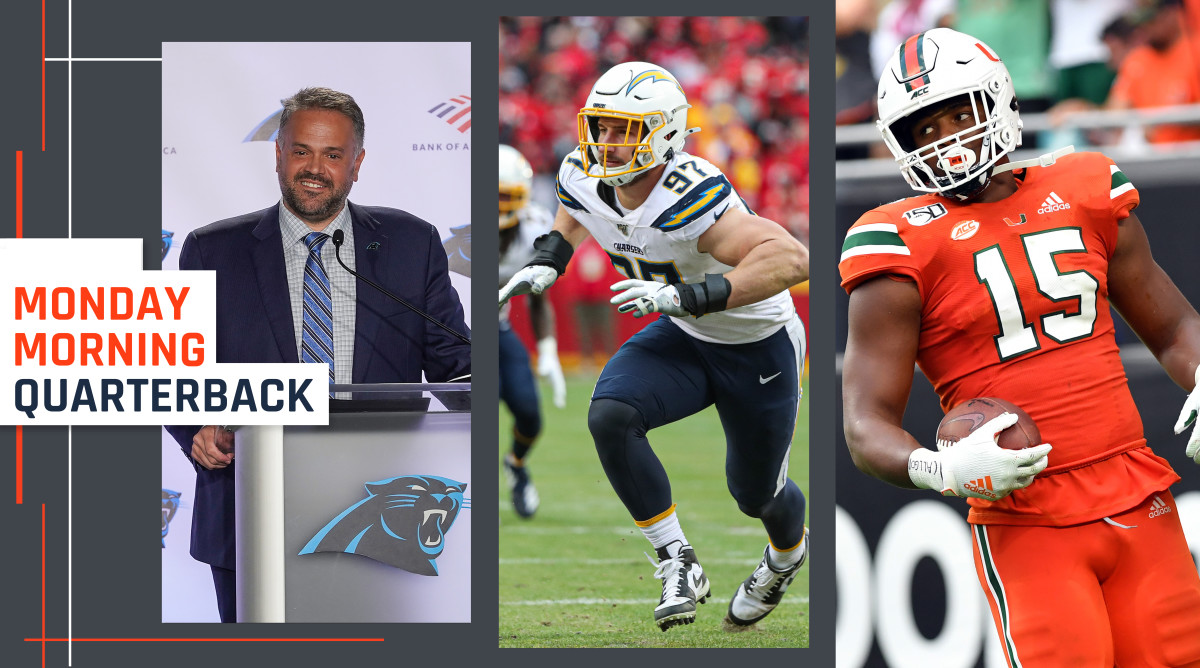The image is a composite collage with distinct sports-related elements and a well-defined structure. On the left, set against a dark gray background, is a man with gray hair and a short gray beard, wearing a blue suit, blue tie, and white checkered shirt, standing at a podium. The podium features a stylized panther logo in black with blue outlines, and the backdrop includes partial text starting with "Bank of America." Moving right, the center image showcases an American football player in navy tights and a white jersey adorned with a yellow lightning bolt with a blue outline, captured mid-run and halfway crouched with arms outstretched, the blurred background implying a stadium atmosphere. On the far right, another football player is clad in a bright orange jersey with green and white shoulder stripes, green tights, white gloves, and a white helmet with green and white stripes, and a red "U" on the side. He is clutching a football to his abdomen. Intersecting red and white lines frame parts of the collage, and a prominent white text box features the text "Monday Morning Quarterback," with "Monday Morning" in orange and "Quarterback" in dark gray.